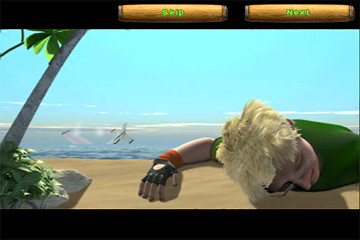This image is a screenshot captured from a cinematic sequence in a video game. The image is framed by black bars at the top and bottom, reminiscent of a widescreen format. On the top black bar, there are two greenish-colored buttons: one on the right that says "Skip" in white font, and one on the left that says "Next" in white font. The scene depicted shows a blonde Caucasian man lying face down on a sandy beach. In the background, there are clear blue skies and a calm ocean. To the left of the man, a small sapling palm tree is visible, bending slightly to the right. The man has scruffy blonde hair, wears glasses, a red shirt, and black gloves.